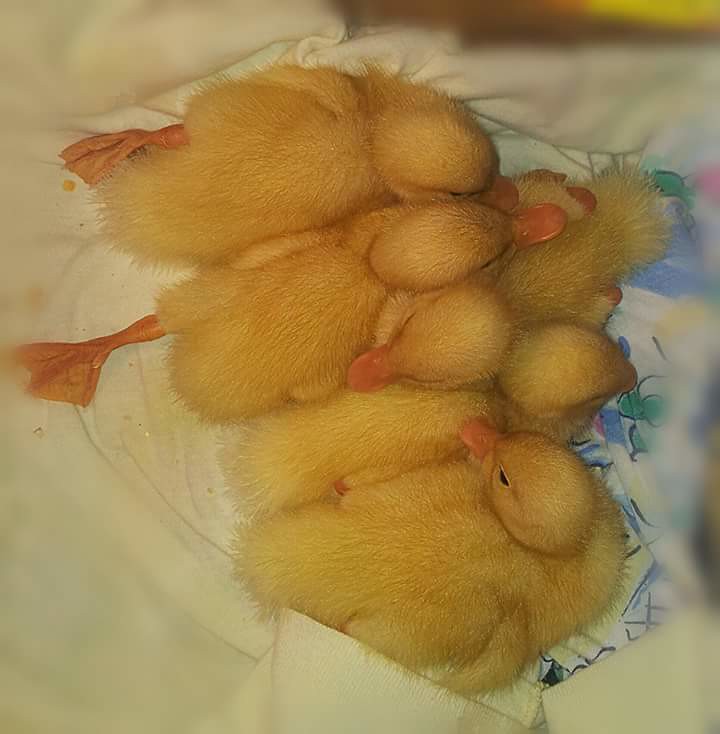This indoor color close-up photograph features a tightly bunched group of approximately seven newly-hatched, bright yellow ducklings seeking warmth from one another. Most of these tiny ducks are nestled on a white blanket or towel adorned with subtle green, pink, blue, and possibly yellow patterns. The ducklings' arrangement has them oriented diagonally, with their tails pointing to the left and their heads mostly to the right, creating a delightful cluster. One standout duckling in the center of the group has its head turned with its bill facing left, in contrast to the others. Noticeably, a portion of another duckling's orange leg is visible mid-left on the image. The scene is well-lit and in focus, capturing the endearing details of their orange bills and the subtle darker hues around the tops of their heads and eyes. Surrounding them is another layer of white fabric, adding to their cozy swaddled appearance.